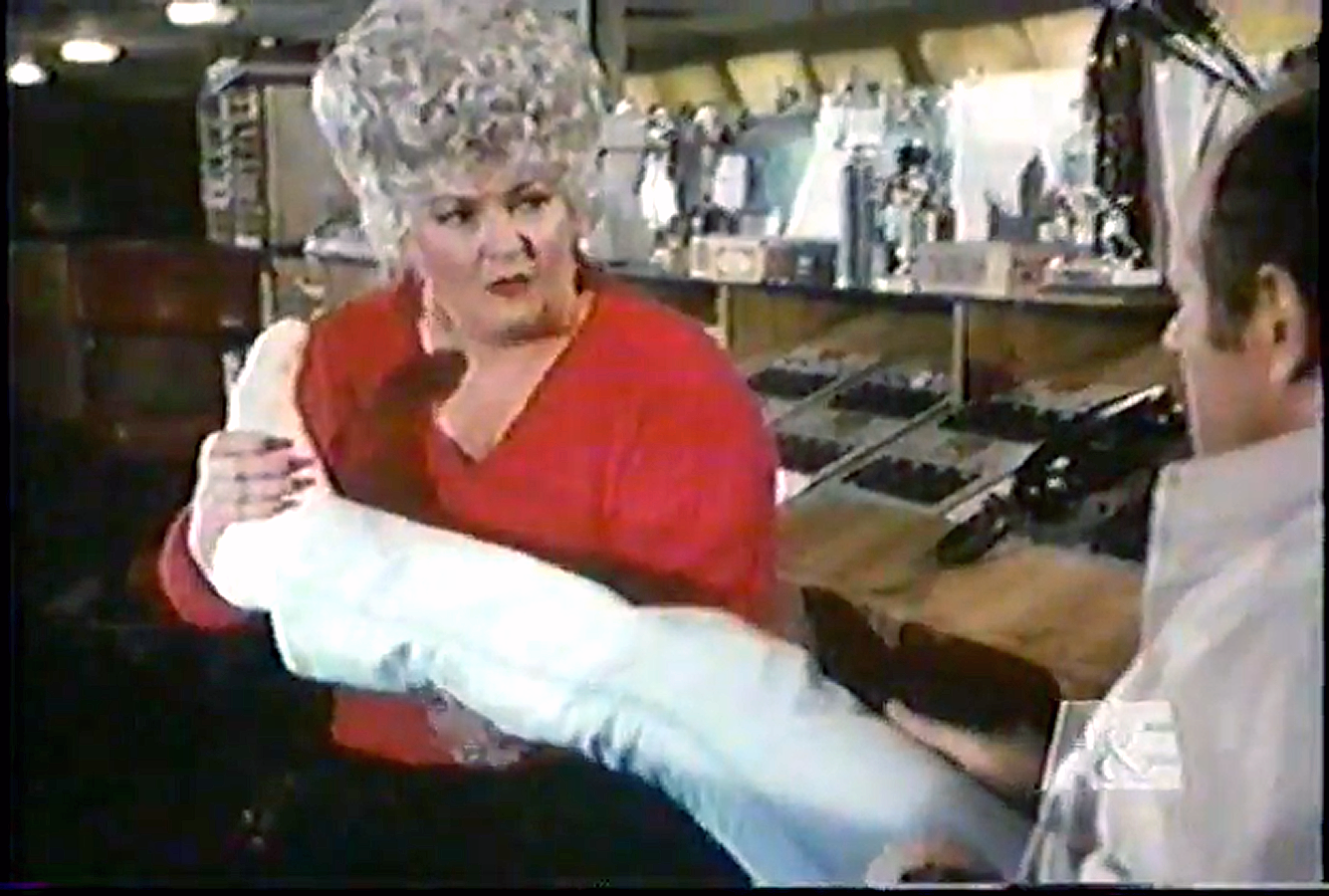The image features a woman standing slightly left of center, facing forward and slightly to the left but turning her head back to the right. She has curly gray or white hair styled high above her head, reminiscent of a not-quite-beehive. She wears a red v-neck sweater and black pants, with the lower part of her body cut off just above the knees. Her right hand is grasping a man's right foot, while her left hand supports his calf. The man, who is partially seen at the bottom right of the image, has short brown hair and wears a light collared shirt, possibly with a wristwatch on his left hand placed on his right thigh. His leg stretches diagonally across the picture. Behind them, a shelf holds various items, including what appears to be a telephone near the man, and a table below bears silver and black objects. In the far background to the left of the woman, an area with dim lighting reveals a chair and ceiling lights. The scene hints at a restaurant setting, indicated by bottles on counters and walls that might be wine bottles.